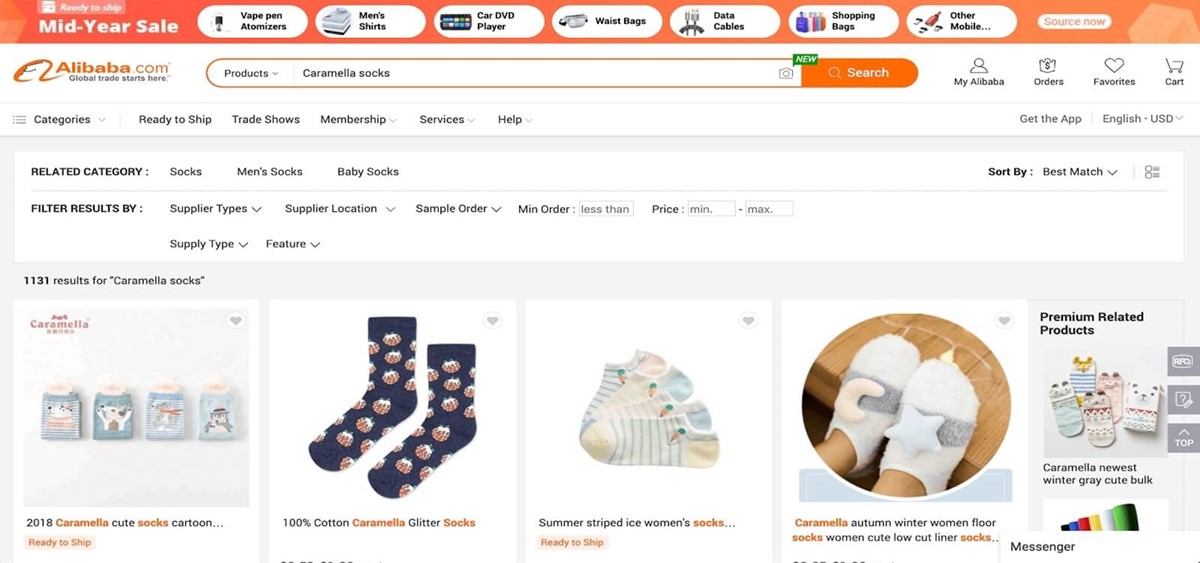**Screenshot of Alibaba Website During Mid-Year Sale**

The screenshot captures the Alibaba website during its Mid-Year Sale. The top of the page features a large orange header with various options displayed in white capsule shapes, each accompanied by a small image illustrating the product category. The options include vape pens and atomizers (with an image of a pen), men's shirts (with a stack of shirts), car DVD players, waste bags like fanny packs, data cables, shopping bags, and mobile accessories. A prominent "Source Now" button is displayed below these options.

In the upper-left corner of the header, the iconic Alibaba.com logo is visible, accompanied by the slogan "Global trade starts here." Adjacent to the logo is a drop-down menu labeled "Products," and the search bar, where "caramella socks" is currently being searched. The search button to the right of the bar is orange. 

To the far right of the header, user navigation options such as "My Alibaba," orders, favorites, and cart are available. Below the header, several categories and options are listed, including "Categories," "Ready to Ship," "Trade Shows," "Membership Services," and "Help." Also, on the right side, there are options to get the app, change the language to English, and convert currency to US dollars.

Additional refined search filters appear, such as supplier types, location, sample order, minimum order, price, supply type, and features. The search results for "caramella socks" yield 1,131 listings, but only five are displayed in the screenshot. Among these are cute baby socks, 100% cotton socks with patterns, summer striped ice women's ankle socks, socks adorned with plush star and moon toys, and another pack of baby socks.